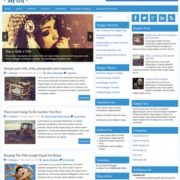A screenshot of a website is presented, featuring a woman biting her nails, adorned with a hat that includes a feather. To the right of the main image, there are five logos. The website is divided into various informational sections, each with blue headers and accompanied by several images and small text. 

One image depicts a wooden rocking chair, another shows what seems to be a bulldozer, and a third, partially cut-off image appears to depict an outdoor scene possibly featuring a ferris wheel or carousel. Additionally, the page includes three more pictures, with the last two in black and white. The overall background of the website is white, contributing to a clean and organized layout.